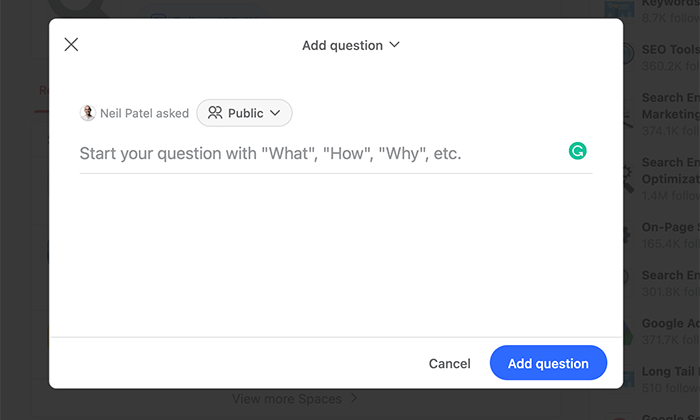The image displays a screenshot of a website interface featuring a prominent overlay box, which occupies the majority of the screen. The overlay box is white and titled "Add Question," accompanied by a dropdown arrow box on the right-hand side. To the left, within this box, there is a clickable 'X' icon indicating an option to close the overlay.

Directly beneath the "Add Question" title, there is an avatar image showing a person's torso, beneath which the text reads "Neil Patel asked." Next to this, a "Public" button is visible, indicating the visibility of the question, and is followed by another dropdown arrow and two small people icons.

Further down, instructional text guides users to start their question with "what," "how," or "why," with these words enclosed in quotation marks followed by "etc." This guidance is placed above a refresh arrow icon, suggesting a clickable option to refresh the content.

Below this instructional text is a blank, white response area where users can type their questions. At the bottom of this response area, a thin gray line separates the main section from the footer options.

In the bottom right-hand corner, the interface provides two buttons: a "Cancel" button and an "Add Question" button. The "Add Question" button is distinctively oval-shaped and blue, poised for users to submit their inquiries.